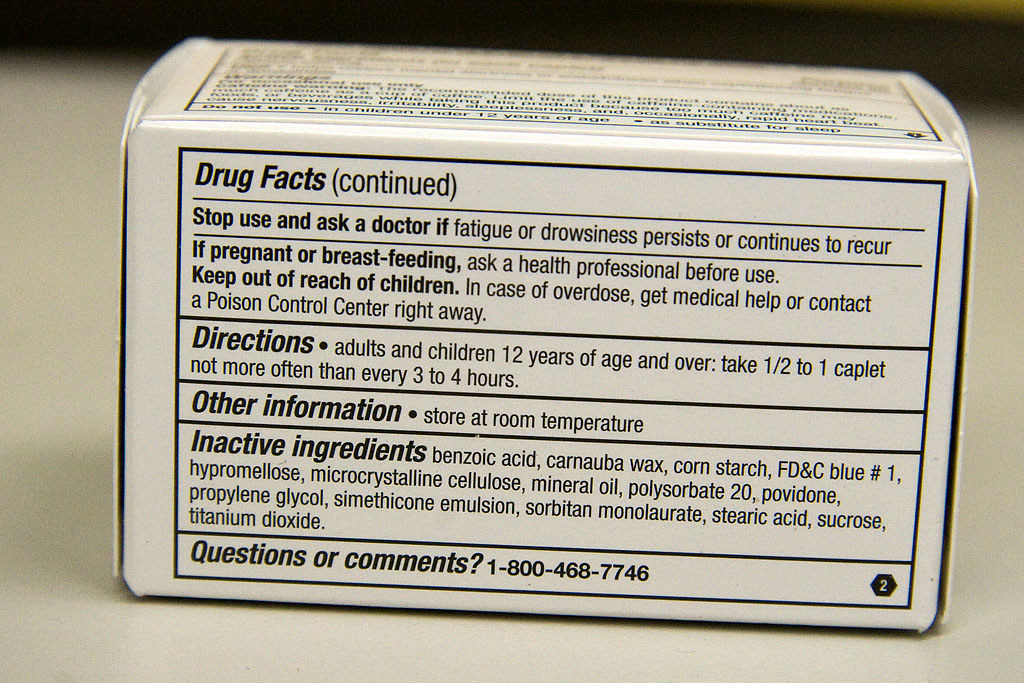The image displays a white, rectangular box of over-the-counter medication resting on a white table. The box features prominently black text on a white background, detailing drug facts. At the top, it reads "Drug facts continued.” It advises to stop use and consult a doctor if fatigue or drowsiness persists or recurs, and to seek medical advice before use if pregnant or breastfeeding. The label warns to keep the product out of reach of children and provides emergency instructions for overdose: get medical help or contact a poison control center immediately.

The directions specify that adults and children aged 12 and over should take half to one caplet no more frequently than every three to four hours. Additional information indicates the product should be stored at room temperature. The inactive ingredients listed include benzoic acid, carnauba wax, cornstarch, FD&C Blue No. 1, hypermellose, microcrystalline cellulose, mineral oil, polysorbate 20, povidone, propylene glycol, simethicone emulsion, sorbitan monolaurate, stearic acid, sucrose, and titanium dioxide.

At the bottom of the box, there is a customer service contact detail, providing a phone number for questions or comments: 1-800-468-7746. In the lower right corner, there is a small number “2” indicating a secondary warning or note within the packaging.